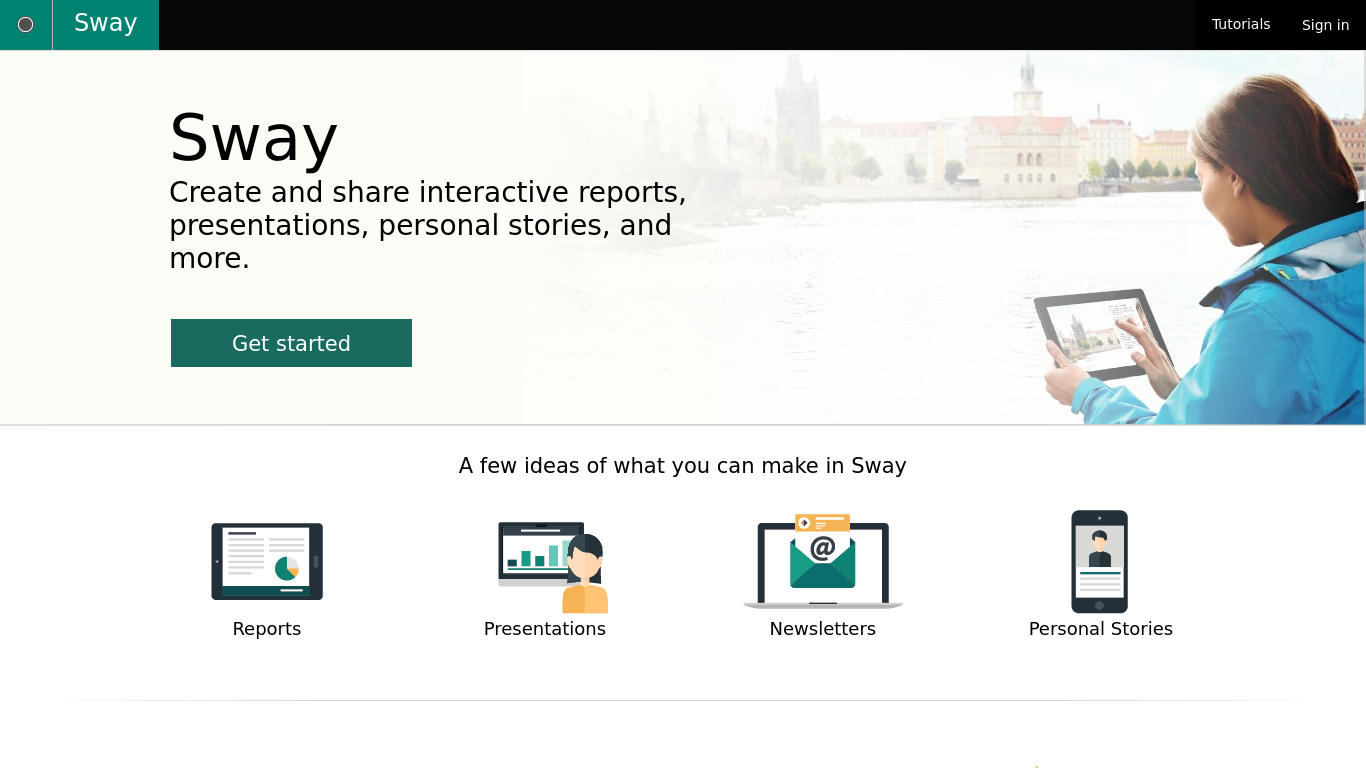This image showcases a web page from the website SWAY. At the top of the screen, there is a thin black banner. A small section at the beginning of the banner is green, featuring the word “SWAY” in white text. Over to the far right of the black banner, you can see the options “TUTORIALS” and “SIGN IN” in tiny white text.

Below the banner, set against a white background, the text "SWAY" is prominently displayed in large black letters. Underneath it, smaller black text reads, "CREATE AND SHARE INTERACTIVE REPORTS, PRESENTATIONS, PERSONAL STORIES, AND MORE." A green button with “GET STARTED” in white text is positioned below this description. To its right, there is an image of a young woman viewed from the side and back, partially in profile. She has long brown hair tucked behind her ear and appears to be smiling at a tablet she is holding, as if about to interact with something on the screen. The background depicts beautiful architecture and trees, suggesting she is in an outdoor setting. Her tablet screen mirrors this scenery. She wears a light blue hooded jacket.

Further down in the middle of the screen, black text declares, "A FEW IDEAS OF WHAT YOU CAN MAKE IN SWAY." Below this headline are four graphics representing different uses: REPORTS, PRESENTATIONS, NEWSLETTERS, and PERSONAL STORIES. Each graphic includes an icon: a document for Reports, a woman standing in front of a screen for Presentations, an email icon for Newsletters, and a cell phone displaying an image of a man for Personal Stories.